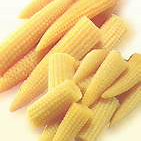The image is a detailed, close-up photograph of a small pile of miniature baby corn arranged on a white background, likely a counter. The corn cobs vary in shape, with some being cylindrical with flat tops and bottoms, while others are more conical, resembling pencils. They are pale yellow with tiny, ridged kernels and some have short stems extending from them. The pile is predominantly oriented towards the lower left corner of the image. Notably, two of the corn cobs on the right side have small black shapes on their tops. The photograph is somewhat grainy, adding to the texture of the corn, and the presence of shadows gives some of the corn a slightly orange hue. The overall impression is that of cut, possibly cooked, baby corn, typical of what could be found in a stir-fry.